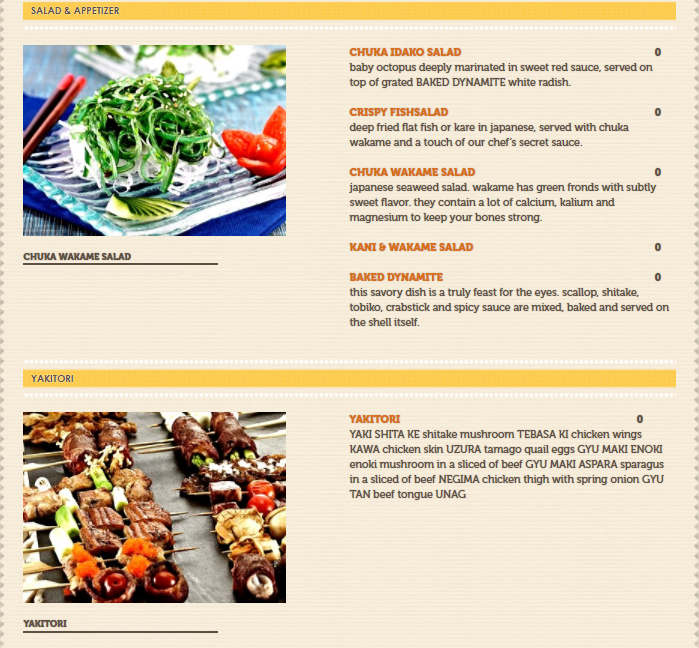The image appears to be a detailed page from a restaurant menu, predominantly featuring Japanese or Asian cuisine. At the top, a yellow header titled "Salad and Appetizer" highlights various dishes, complemented by vivid images on a light brown, paper-like digital background. Prominently featured is the Chuka Wakame Salad, a Japanese seaweed salad known for its green fronds and subtly sweet flavor, rich in calcium, magnesium, and potassium.

The menu includes:
- **Chuka Idiko Salad**: Baby octopus deeply marinated in a sweet red sauce, served on top of grated, baked dynamite white radish.
- **Crispy Fish Salad**: Deep-fried flatfish, or 'kare' in Japanese, served with Chuka Wakame and a touch of the chef's secret sauce.
- **Chuka Wakame Salad**: Japanese seaweed salad with a delicate flavor, known for its nutritious benefits.
- **Kani and Wakame Salad**: Although not described in detail, likely features crab and seaweed.
- **Baked Dynamite**: A visually appealing dish with scallops, shiitake mushrooms, tobiko, crab stick, and spicy sauce, mixed, baked, and served in the shell.

Below these sections, a yellow divider labeled "Yakitori" introduces a variety of skewered meats and vegetables:
- **Yakitori Selections**: This includes shiitake mushrooms, chicken wings (tibasaki), chicken skin (kawa), tamago (quail eggs), enoki mushrooms wrapped in sliced beef (gyu-maki), asparagus in sliced beef (gyu-maki), and chicken thighs with spring onion (negima), among others.

The overall composition of the menu is visually appealing, designed with colorful images and descriptive text that elaborate on the nutritious and flavorful offerings.